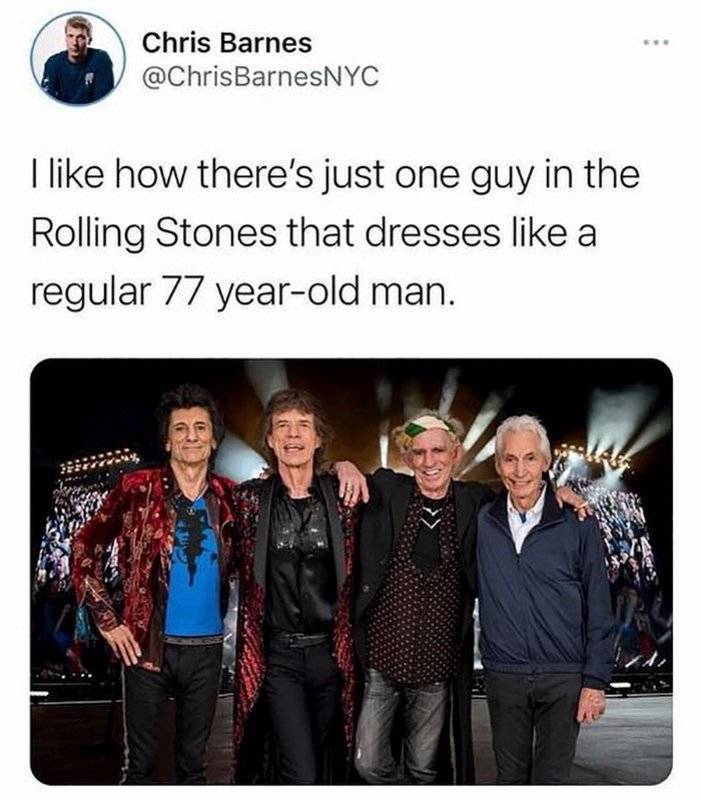The image depicts a screenshot of a social media post from a user named Chris Barnes, who is identified by a profile picture showing a man with short blonde hair wearing a blue jumper. At the top of the screen, it says "Chris Barnes, NYC," and the accompanying tweet reads, "I like how there's just one guy in the Rolling Stones that dresses like a regular 77-year-old man." Below the text is a rectangular, rounded-edged image of the Rolling Stones standing on a stage. The band members, four elderly men, are positioned centrally and are facing the camera, smiling. They are flanked by screens displaying a nighttime crowd and stage lights. On the far left, one man with black hair wears a red jacket over a blue shirt with black pants. Next to him, a man with long brown hair wears a red blazer and a black shirt. Beside him, another man sports a black jacket, a waistcoat with white dots, and washed-out black jeans, with a striped green and yellow band around his head. On the far right, the final man with light gray hair is dressed in a plain blue zip-up jacket and gray trousers or jeans. The scene captures the band in an informal pose, highlighting a contrast in their attire, which aligns with Chris Barnes' humorous observation in the tweet.